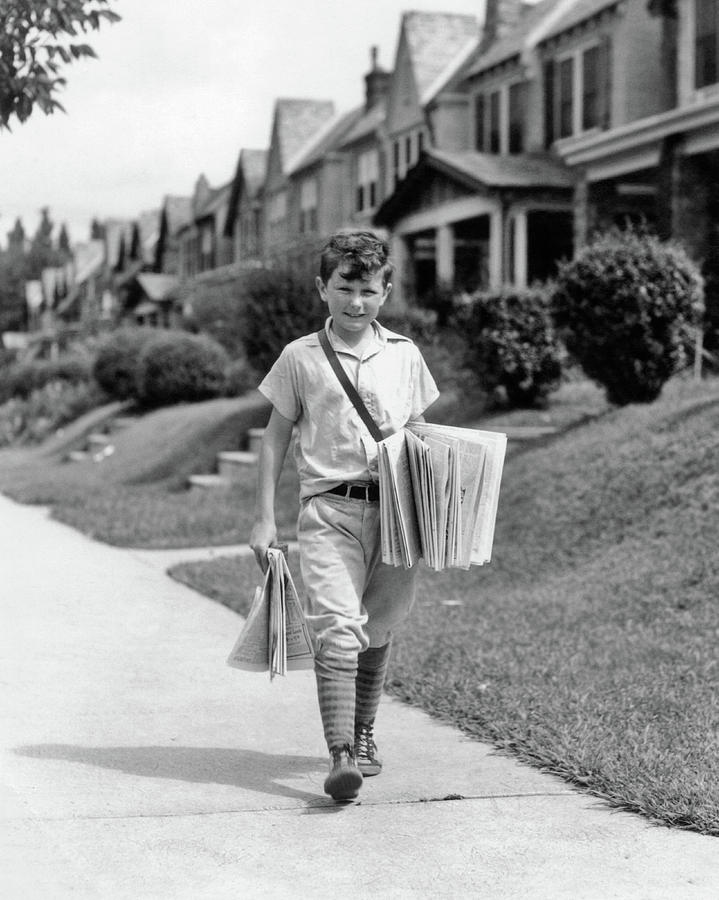This black and white photograph, rectangular in shape with its long sides on the left and right, captures a nostalgic outdoor scene set in the 1930s or 1940s. Occupying the center of the image is a young boy, approximately seven or eight years old, walking down a diagonally positioned sidewalk that stretches from the mid-left to the lower right. He is evidently a paperboy, as indicated by the stack of newspapers tucked under one arm and a single newspaper held in his other hand. The boy is dressed in traditional attire of the era: a short-sleeved collared shirt, a pair of light-colored pants secured with a black belt, and long striped socks paired with black lace shoes. A satchel bag crosses his chest, further emphasizing his role.

He appears to be smiling faintly as he makes his way towards the camera. Behind him, a grassy slope ascends towards a row of two-story houses, complete with traditional angled roofs and stone steps that lead up from the sidewalk. Shrubs dot the small front lawns, adding to the quaint, residential charm of the scene. The overall composition of the photograph, with its detailed depiction of the young paperboy and the surrounding suburban neighborhood, paints a vivid picture of a bygone era.